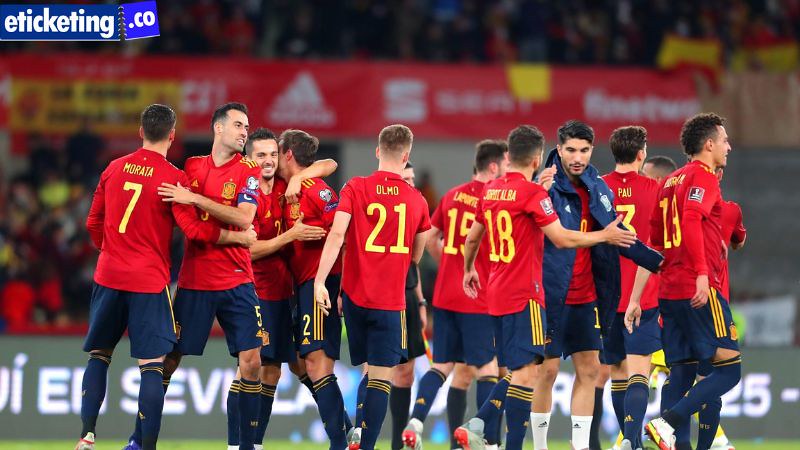The image captures the jubilant moment of a soccer team celebrating after their match, with players engaging in various expressions of camaraderie such as hugging, high-fiving, and shaking hands. The team members are clad in red tops featuring white lettering and various numbers including 3, 7, 13, 15, 18, and 21. Most players are also wearing long blue socks adorned with yellow stripes, except for one player donning white socks. They complete their uniforms with blue shorts and blue shin guards. In the background, a densely packed stand is visible, highlighted by a long red Adidas advertisement, identifiable by its white logo despite the blur. There's also an ad for e-ticketing.co visible in the top corner. A man in a jacket, possibly the coach, is also present, adding another layer of detail to the vibrant scene.